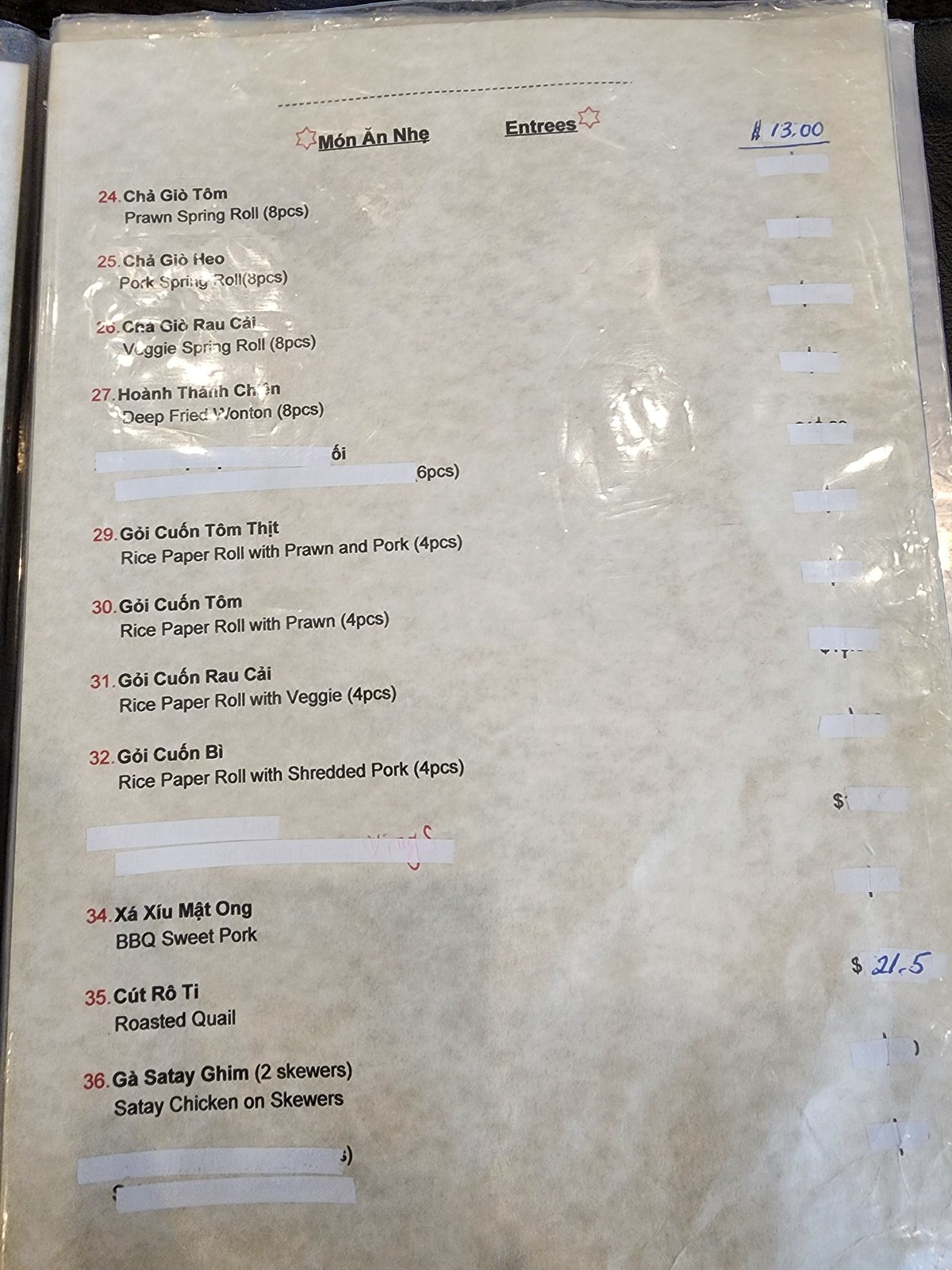This photograph captures a detailed image of a piece of paper encased in a protective plastic cover. The document appears to be a menu, likely from a Chinese or Taiwanese restaurant, as the text is written in what seems to be an Asian language. The top of the menu features the words "Mone and Nay," which likely indicates "Entries."

The menu is organized into columns; the first column lists the menu numbers, written in conspicuous red ink, while the rest of the descriptions and prices are in black. Item number 24, labeled as "Jing," is described as prawn spring rolls, and appears to have its price obscured by white-out, though it is inferred to be $13.

Subsequent items include:
- Number 25: Pork spring rolls (8 pieces)
- Number 26: Veggie spring rolls (8 pieces)
- Number 27: Deep-fried wontons (8 pieces)
- Number 29: Rice paper rolls with prawn and pork (4 pieces)
- Number 30: Rice paper rolls with prawns (4 pieces)
- Number 31: Rice paper rolls with veggies (4 pieces)
- Number 32: Rice paper rolls with shredded pork
- Number 34: Barbecue sweet pork

Additionally, the menu transitions into meal options, starting with item number 34 and listing as:
- Number 36: Chicken (priced at $21.50)

The use of red and black ink creates a visual hierarchy, distinguishing meal numbers from descriptions and prices. The overall layout and detailed descriptions suggest a diverse offering of spring rolls, wontons, and rice paper rolls that cater to various dietary preferences.